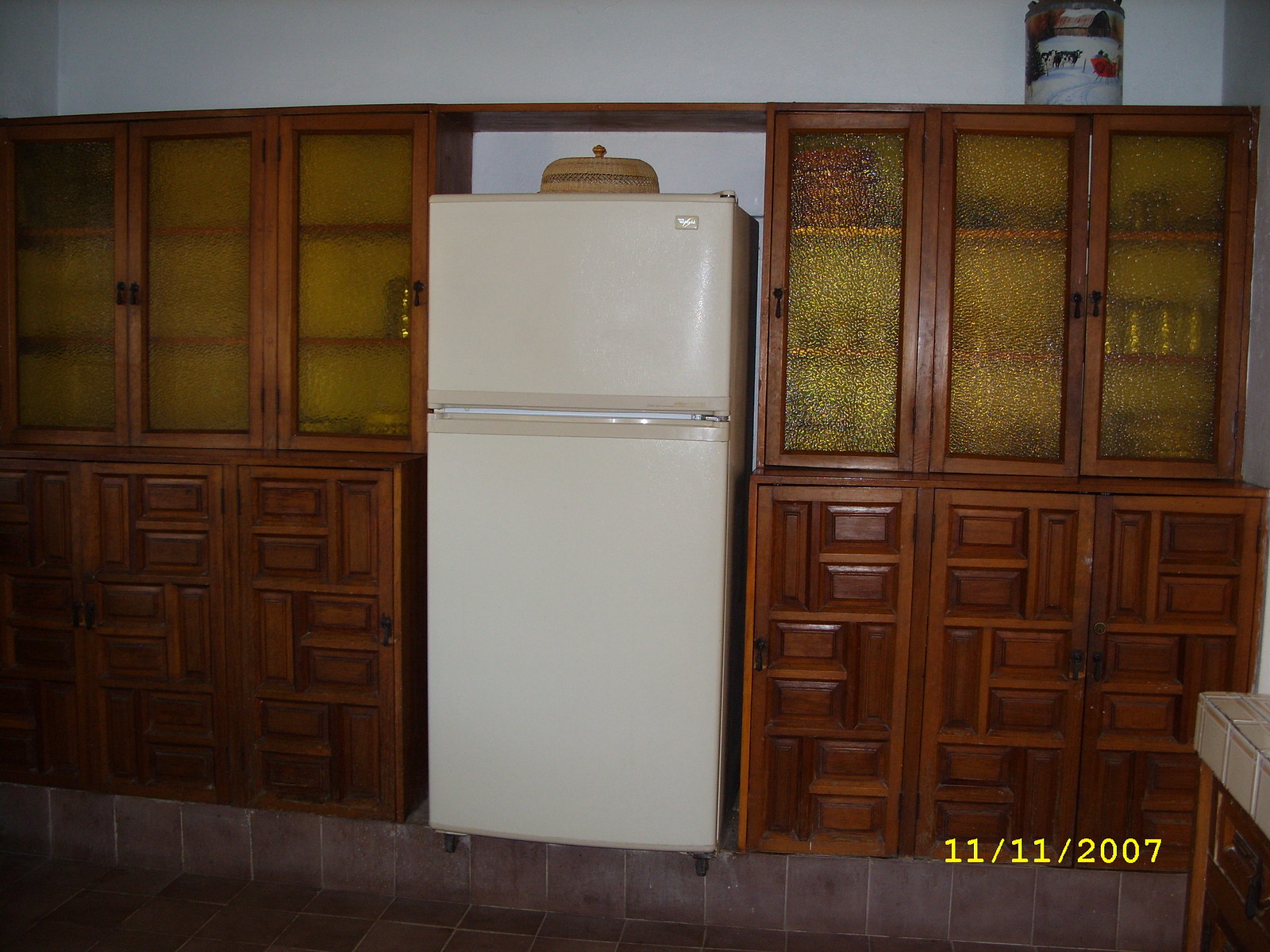This photograph, dated 11-11-2007 in the lower right-hand corner in yellow font, showcases a charmingly vintage kitchen that appears older than its timestamp. The kitchen features brick flooring which extends upward by about 6-8 inches to form a ledge. Centrally placed on this ledge is an older-looking, almond-colored refrigerator with a top freezer that occupies about one-third of the appliance's height. Resting atop the refrigerator is a wicker basket with a tan lid featuring black detailing, possibly used for bread storage.

Flanking the refrigerator on both sides are built-in wooden cabinets, their deep medium-brown doors adorned with rectangular carvings. The upper cabinets feature slightly opaque, yellowish-tan glass doors that swing open from alternating sides, behind which faintly discernible cups, glasses, and canned goods are stored. At the very top of the cabinets sits a tall canister with a wintry scene depicting cows and a red sleigh, suggesting it might be a holiday popcorn tin.

The overall ambiance of the kitchen, from its Mediterranean-inspired brick floor to the detailed vintage cabinetry, suggests a timeless charm that belies the 2007 date.